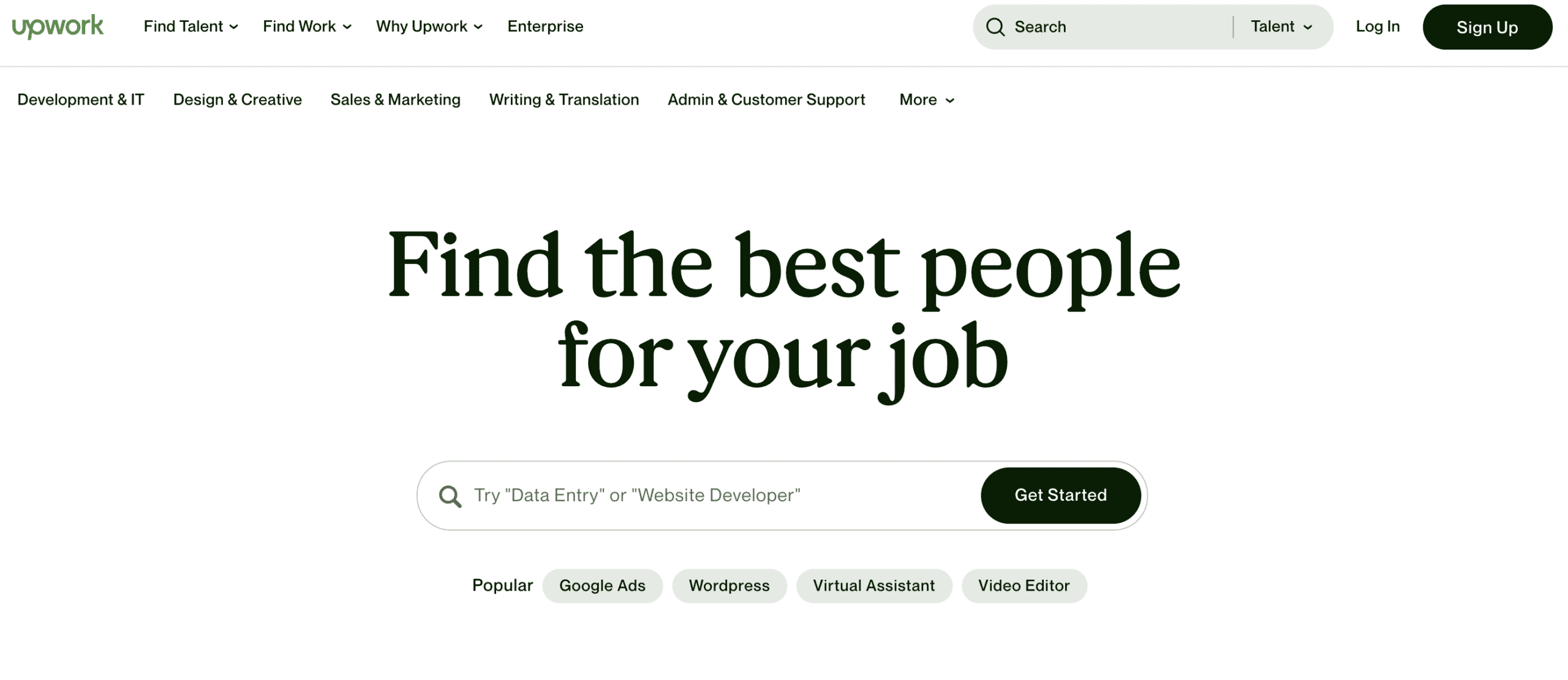The image showcases the homepage of the Upwork website, a popular online platform for freelancers and clients to connect. The Upwork logo, written in green, is prominently displayed at the top. Below the logo, the main navigation bar includes drop-down menus for different sections: "Find Talent," "Find Work," "Why Upwork," and "Enterprise."

Beneath the navigation bar, a sub-menu features categories such as "Development & IT," "Design & Creative," "Sales & Marketing," "Writing & Translation," "Admin & Customer Support," and more.

On the top right side, there is a search bar labeled "Search Talent," alongside login and sign-up buttons; the latter is highlighted in dark green.

Central to the image is the bold tagline "Find the Best People for the Job," set against a white background. Directly underneath, another search bar suggests options like "Data Entry" or "Website Developer." Adjacent to this search bar is a dark green "Get Started" button.

At the bottom of the page, popular tags such as "Popular," "Google Ads," "WordPress," "Virtual Assistants," and "Video Editors" are listed, indicating commonly sought-after skills on the platform. The overall theme of the website combines green and dark green text against a clean, white background.